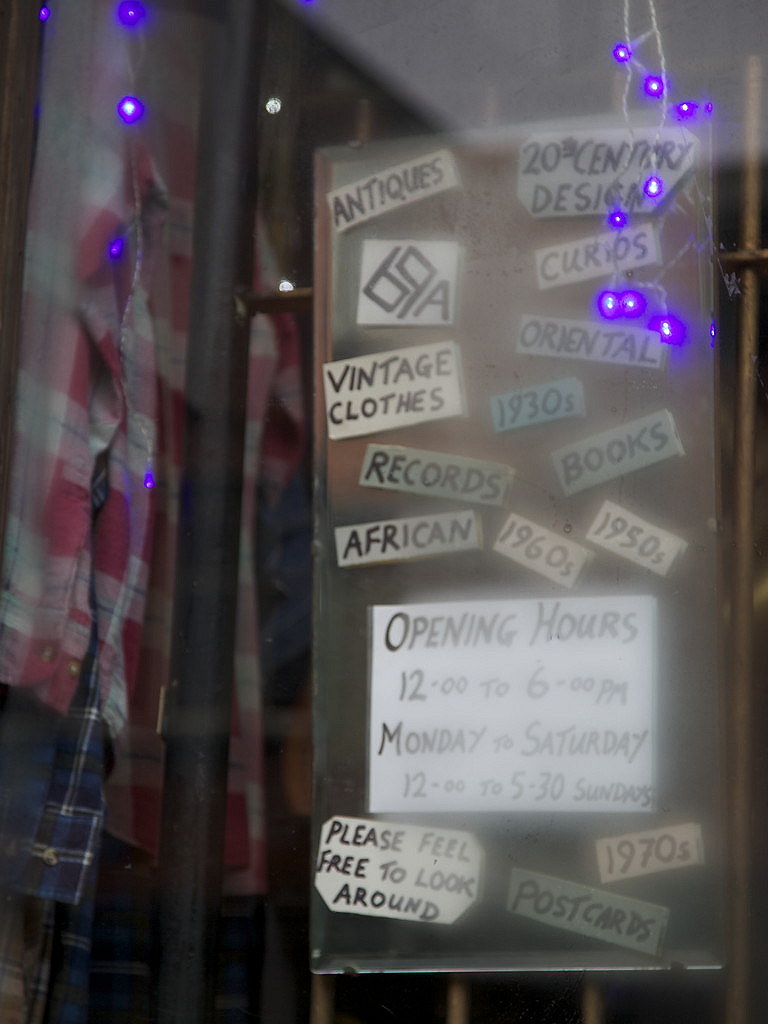The photograph depicts a vintage store's window display with a prominent tall rectangular wooden board, positioned behind glass. Attached to this wooden board are various pieces of paper, each advertising different items such as "Antiques," "20th Century Design," "Oriental," "1930s," "Vintage Clothing," "Books," "Records," "African," "1960s," and "1950s." Central to the display is a large white paper detailing the store's opening hours: "12 PM to 6 PM, Monday to Saturday," and "12 PM to 5:30 PM on Sundays." Below this, additional signs mention "1970s," "Postcards," and an invitation for customers to "Please feel free to look around." Completing the scene, there are plaid shirts and what appear to be tablecloths or fabrics positioned on either side of the window, along with a string of LED lights, contributing to the vintage aesthetic.